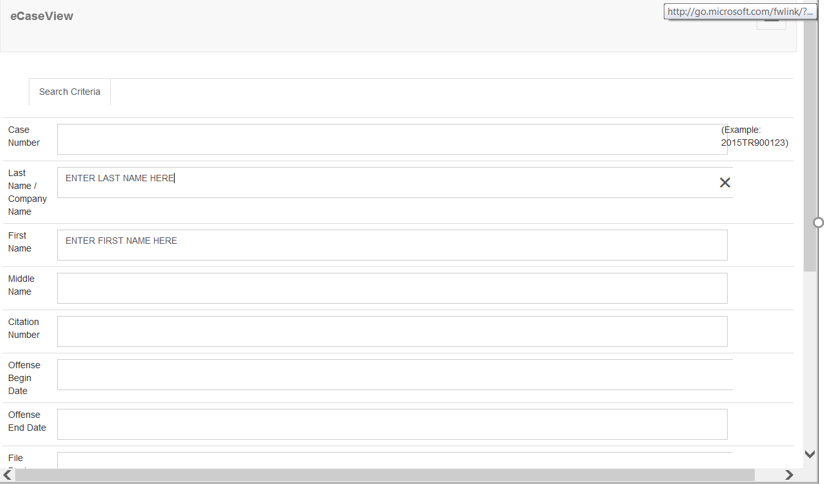The image depicts a detailed form interface with various input fields, each designed for specific data entries. In the upper left-hand corner, the label "E CASEVIEW" is prominently displayed. On the upper right-hand side, there's a URL link: go.microsoft.com/FWLIKNK.

The form consists of many rows, each separated by distinct sections. The background color of the form is primarily white, with the exception of the first stripe at the top, which has a light gray background.

Starting with the top row, it is labeled "Search Criteria," serving as the header for the form. The layout is organized into two columns: the left column contains labels for each entry, and the right column provides the corresponding text fields where users are required to enter information.

Below the "Search Criteria" header, the first row has the label "Case Number" on the left, with an example input "2015 TR 900123" on the right. The following row asks for the "Last Name / Company Name," instructing users to enter the last name or company name.

Subsequently, the form requests:
- "First Name" where users enter the first name.
- "Middle Name" where users enter the middle name.
- "Citation Number" which requires the citation number.
- "Offense Begin Date" and "Offense End Date" where users need to input the respective dates.

Each of these fields must be manually filled in by the user. Additionally, on the far right, stretching from the upper right to the lower right, there is a menu pull-down stripe, perhaps for additional settings or options related to the form.